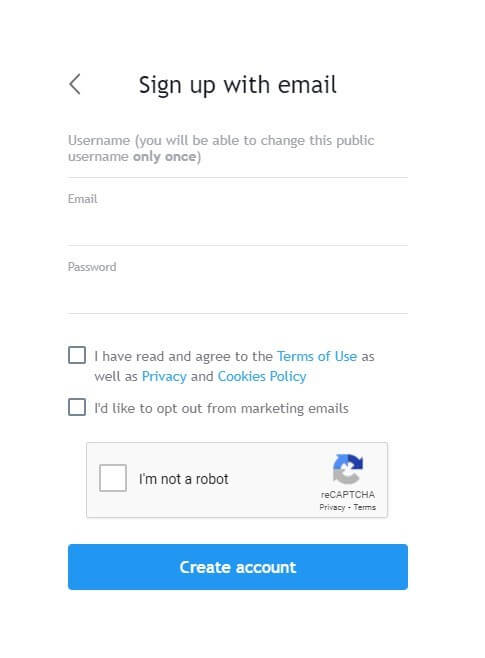A detailed screen capture showcasing a sign-up form on a mobile device, outlined in a clean, user-friendly layout. The form prompts the user to provide essential registration information, including a public username (modifiable only once), email address, and password. Below these fields, there are two checkboxes for agreeing to the Terms of Use and Privacy and Cookies Policy, with clickable links for each policy, highlighted in blue. Users also have the option to opt out of marketing emails by selecting an additional checkbox. To ensure security, there's a reCAPTCHA verification box labeled "I'm not a robot," accompanied by links to the reCAPTCHA Privacy and Terms of Service. The process is completed by clicking the prominent blue "Create Account" button at the bottom of the form.